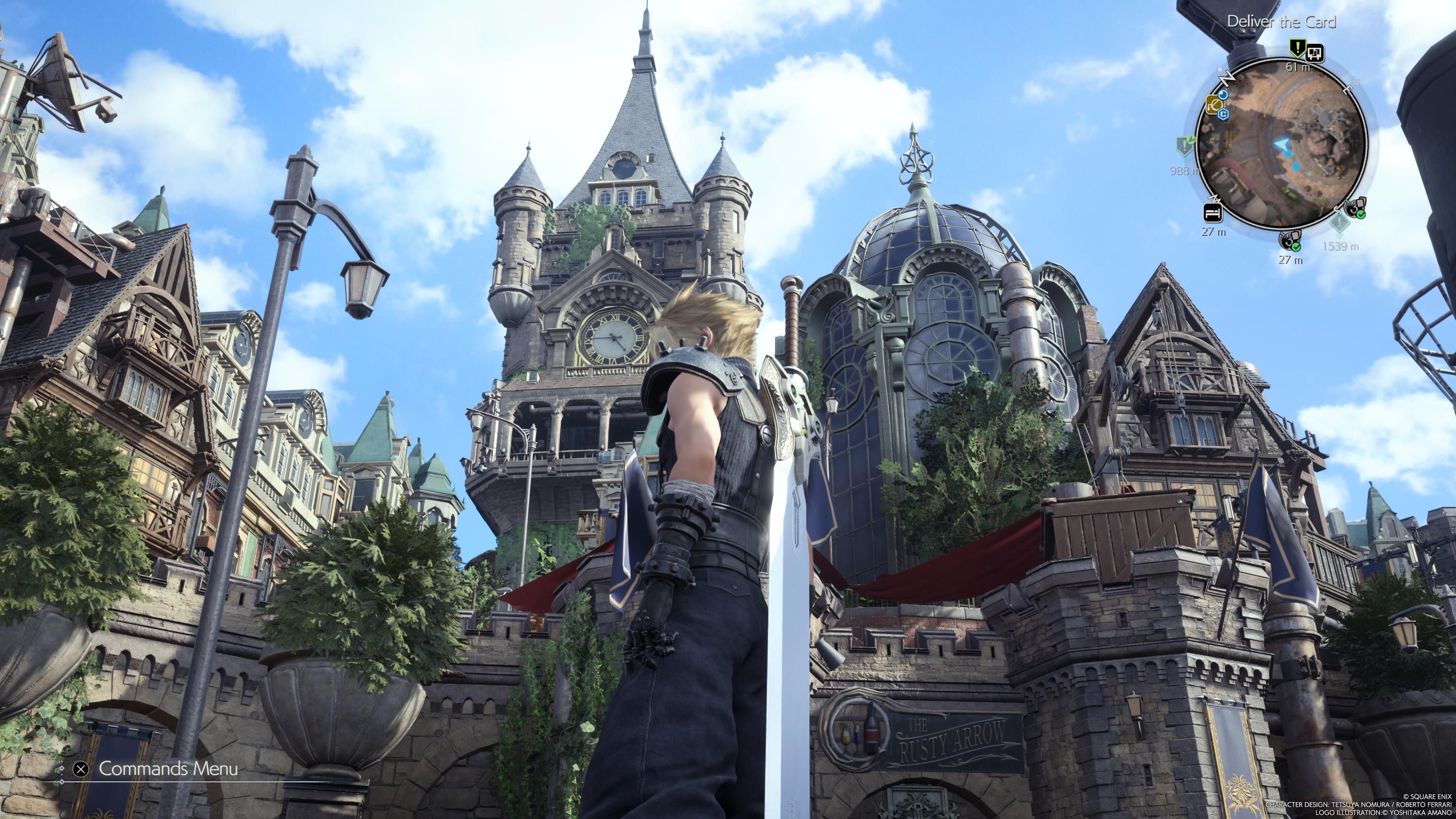The image is a detailed screenshot from a fantasy RPG video game, showcasing a highly realistic and vivid medieval village scene. At the center foreground stands a muscular character with blonde hair, equipped with black gloves, a black uniform, and a large sword strapped to their back. The character is positioned in front of a striking building that combines elements of both Gothic and steampunk architecture, prominently featuring a large, pointy clock tower. This building is likely some form of cathedral or castle. 

In the top right corner of the screen, there is an in-game overlay displaying a mini-map and a quest directive labeled "Deliver the Card." The bottom left corner shows text labeled "command menus," suggesting that this is indeed a video game interface. The village itself is filled with medieval-style buildings of varying shades of light gray and brown, adorned with flags and archways. Streetlights and stylized lampposts add to the ambiance, along with large planters brimming with green foliage. The sky overhead is a light blue, dotted with white clouds, completing the scene's immersive, old-world charm.